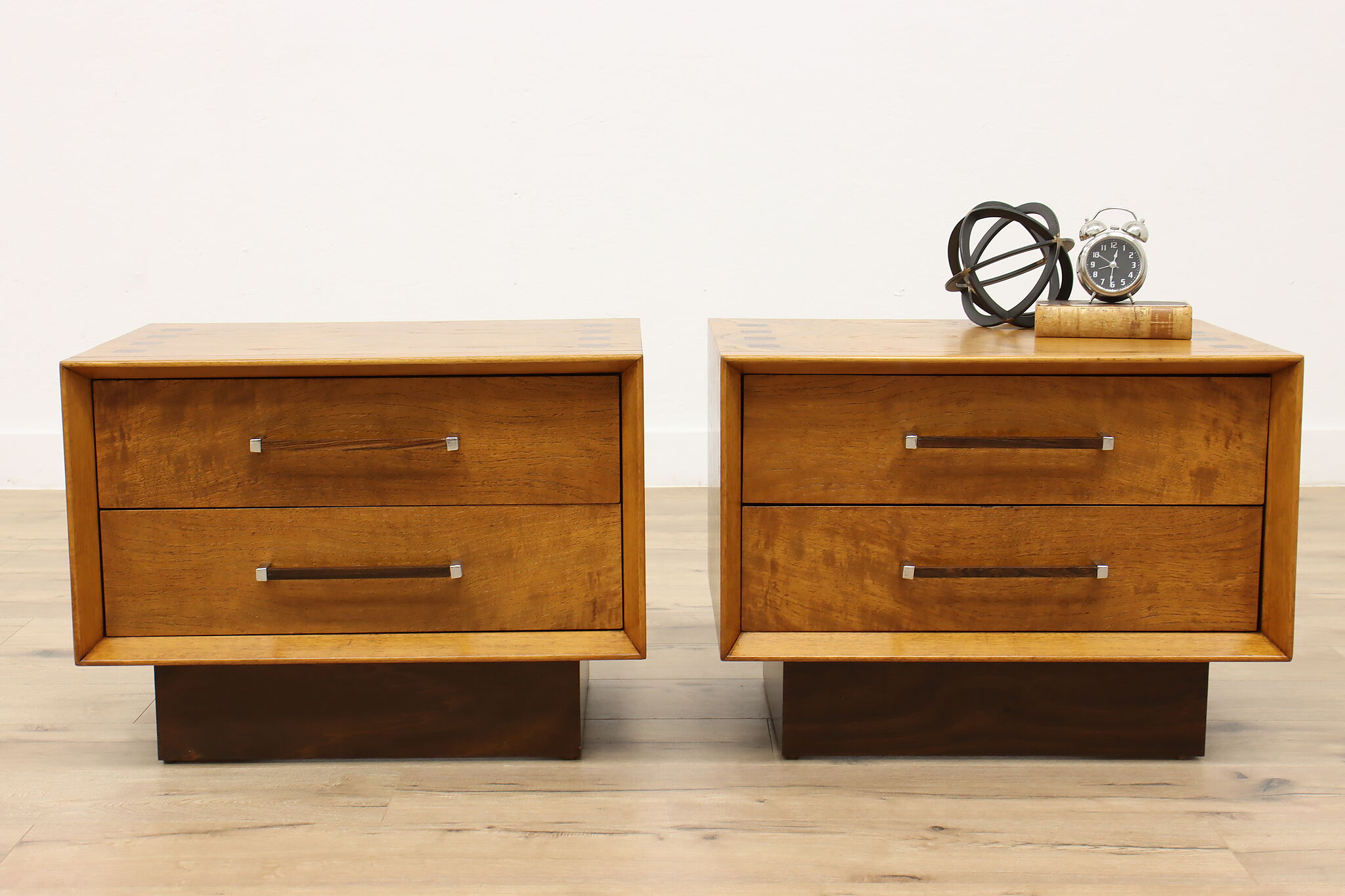This detailed color photograph captures two identical wooden dressers, each with two recessed shelves enclosed by sloped boundaries. The grain of the light brown wooden floor beneath them runs horizontally from left to right, leading to a stark white wall in the background. Both dressers rest on smaller, darker brown rectangular platforms that add a complementary contrast to the lighter wood of the main dresser bodies. Each shelf is fitted with long, narrow wooden handles, secured by small metal squares.

Notably, the dresser on the right features several objects on its top surface. A book lays prominently, accompanied by a silver metal alarm clock with a black face, indicating the time as 12:50. Additionally, there is an intriguing black round object composed of three interconnected circles.